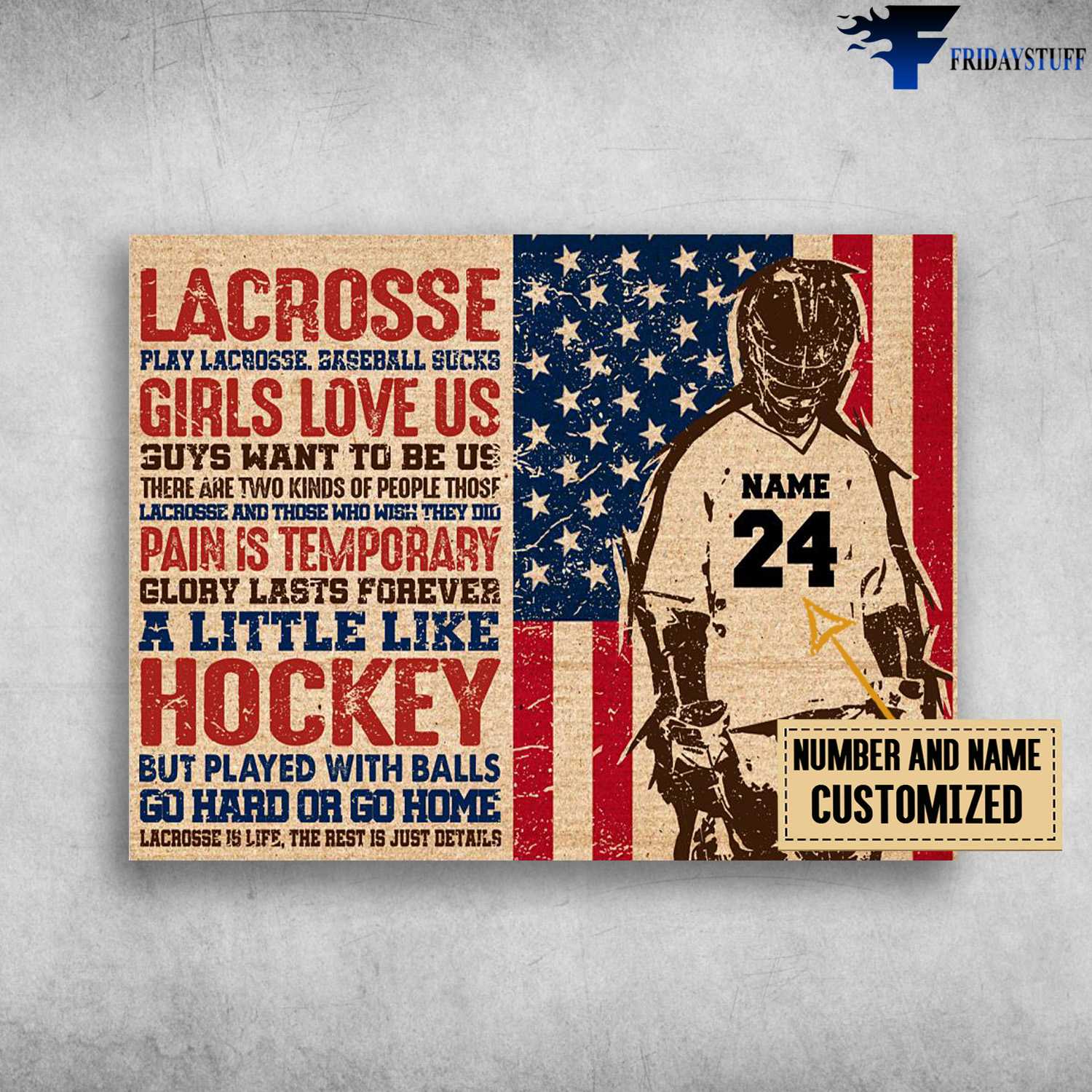This image is an advertisement poster for lacrosse, prominently featuring motivational text in red, white, and blue colors on the left side. It highlights slogans such as "Lacrosse, play lacrosse," "Girls love us, guys want to be us," "There are two kinds of people, those who play lacrosse and those who wish they did," "Pain is temporary, glory lasts forever," "A little like hockey but played with balls," and "Go hard or go home." The text also reads "Lacrosse is life; the rest is just details."

On the right side of the poster, there is an American flag with the stars positioned to the left and the stripes running vertically. In front of the flag stands the silhouette of a person wearing a lacrosse jersey labeled "Name" with the number "24." An arrow beneath the image points to the customizable area on the shirt that reads "number and name customized," indicating the option for personalized jerseys.